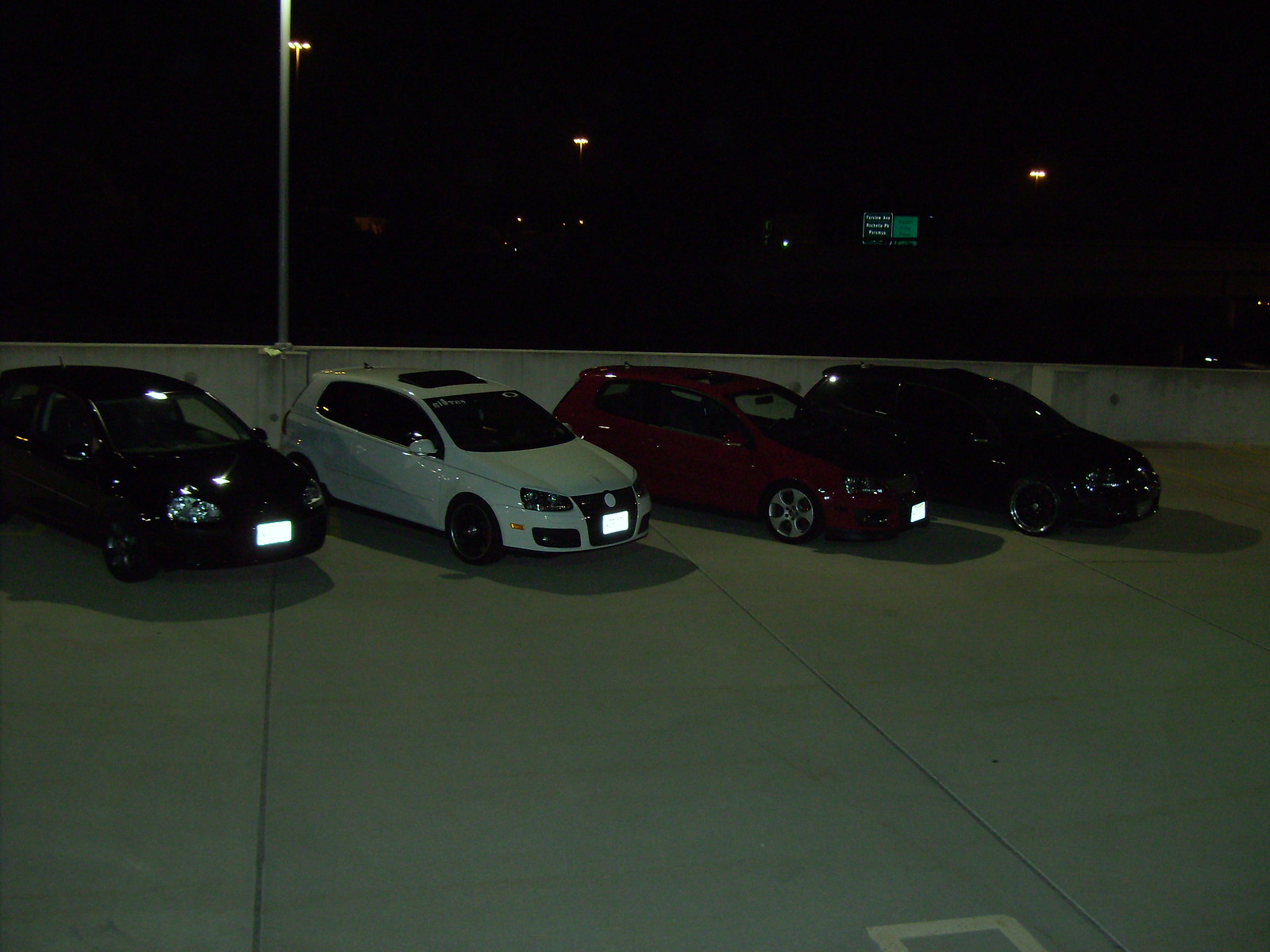The image is a nighttime color photograph capturing a scene on what appears to be the top floor of a multi-storey parking structure. Due to the low light conditions and the cropping of the photograph, the exact location is indeterminate. The scene shows four vehicles parked at an angle, with the front of each vehicle pointing toward the front right diagonal. The front license plates of the first three vehicles from the left reflect the camera's flash prominently. All vehicles appear to be hatchbacks, with the one in the center being white and equipped with a sunroof, while the others are black and maroon. 

The photograph is dimly lit, likely illuminated by an off-frame light source such as a street lamp. In the background, a low wall runs at about the height of a vehicle roof. The concrete floor is segmented into large block slabs with visible vertical lines between them. Scattered small specks of light dot the background, likely distant streetlights, further hinting at an urban environment. On the left side of the image, attached to the wall behind the vehicles, stands a slightly illuminated grey or silver pole, probably a light pole. The backdrop fades into darkness, with only glimmers of light indicating the distant cityscape and a faint green billboard barely visible.